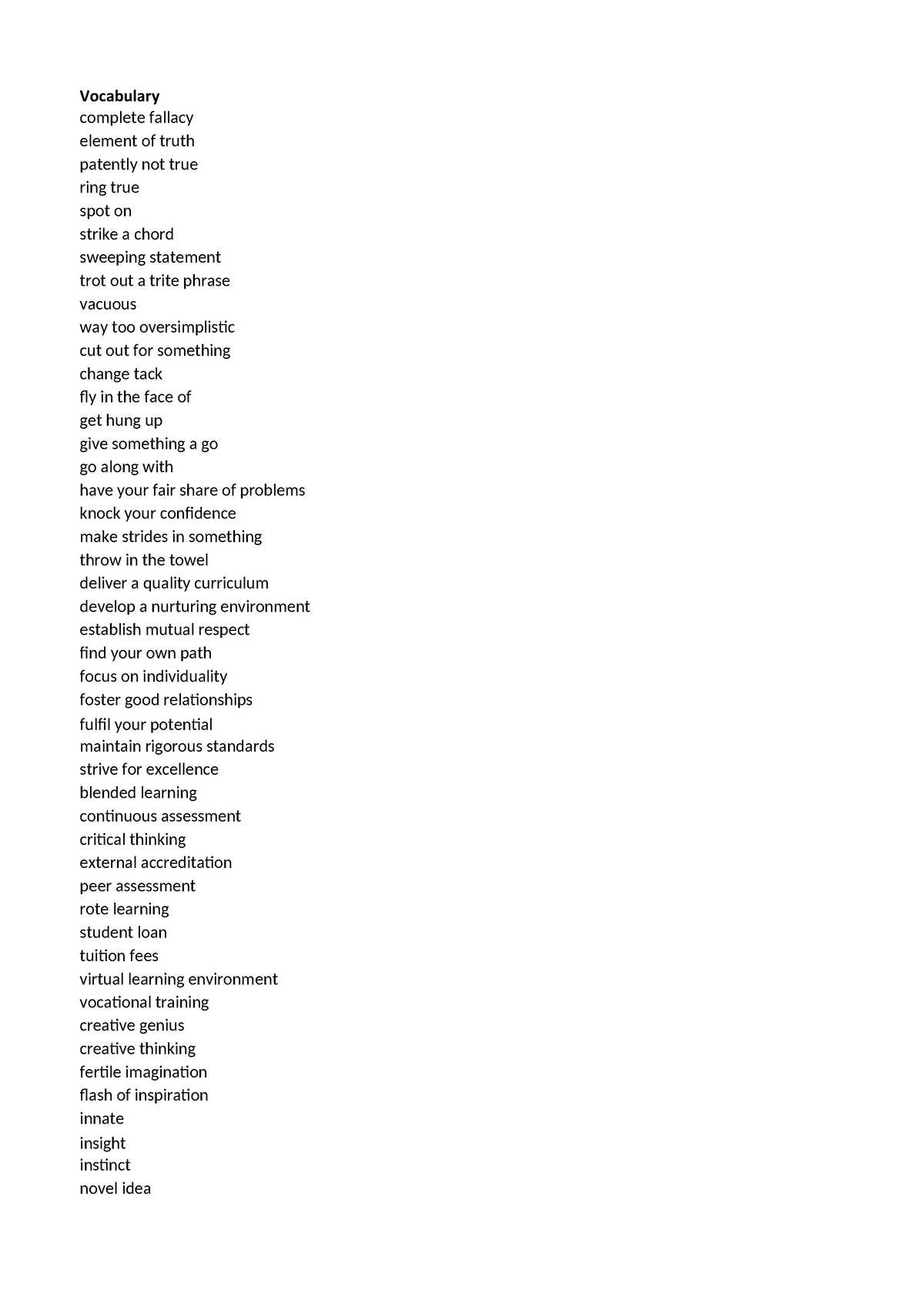The image presents an array of black text on a white background, organized into several horizontal rows. The text is primarily a vocabulary list, comprised of various phrases and terms. Starting from the top, it features words and expressions such as: "vocabulary," "complete fallacy," "element of truth," "patently not true," "ring true," "spot on," "strike a chord," "sweeping statement," "trot out a trite phrase," "vacuous," "way too over simplistic," "cut out for something," "change tack," "fly in the face of," "get hung up," "give something a go," "go along with," "have your fair share of problems," "knock your confidence," "make strides in something," "throw in the towel," "deliver a quality curriculum," "develop a nurturing environment," "establish mutual respect," "find your own path," "focus on individuality," "foster good relationships," "fulfill your potential," "maintain rigorous standards," "strive for excellence," "blended learning," "continuous assessment," "critical thinking," "external accreditation," "peer assessment," "rote learning," "student loan," "tuition fees," "virtual learning environment," "vocational training," "creative genius," "creative thinking," "fertile imagination," "flash of inspiration," "innate," "insight," "instinct," and "novel idea."

The text appears to be a comprehensive compilation aimed at enhancing one's lexicon with a focus on educational terminologies, motivational phrases, and concepts tied to individual growth, learning environments, and creative thinking.